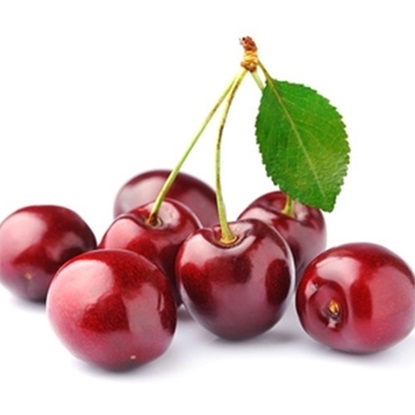The image depicts seven bright red cherries with a shiny, enamel-like gloss. Three of the cherries are connected by their stems, which feature a single green leaf. The other four cherries are detached from their stems and lie scattered around. The cherries appear fresh and ripe, exhibiting a mix of light and dark red hues, with some showing darker spots. They are positioned on a plain white background, possibly a table or cloth, against which their vivid coloration stands out. The entire image is devoid of text, people, or additional objects, focusing solely on the cherries.